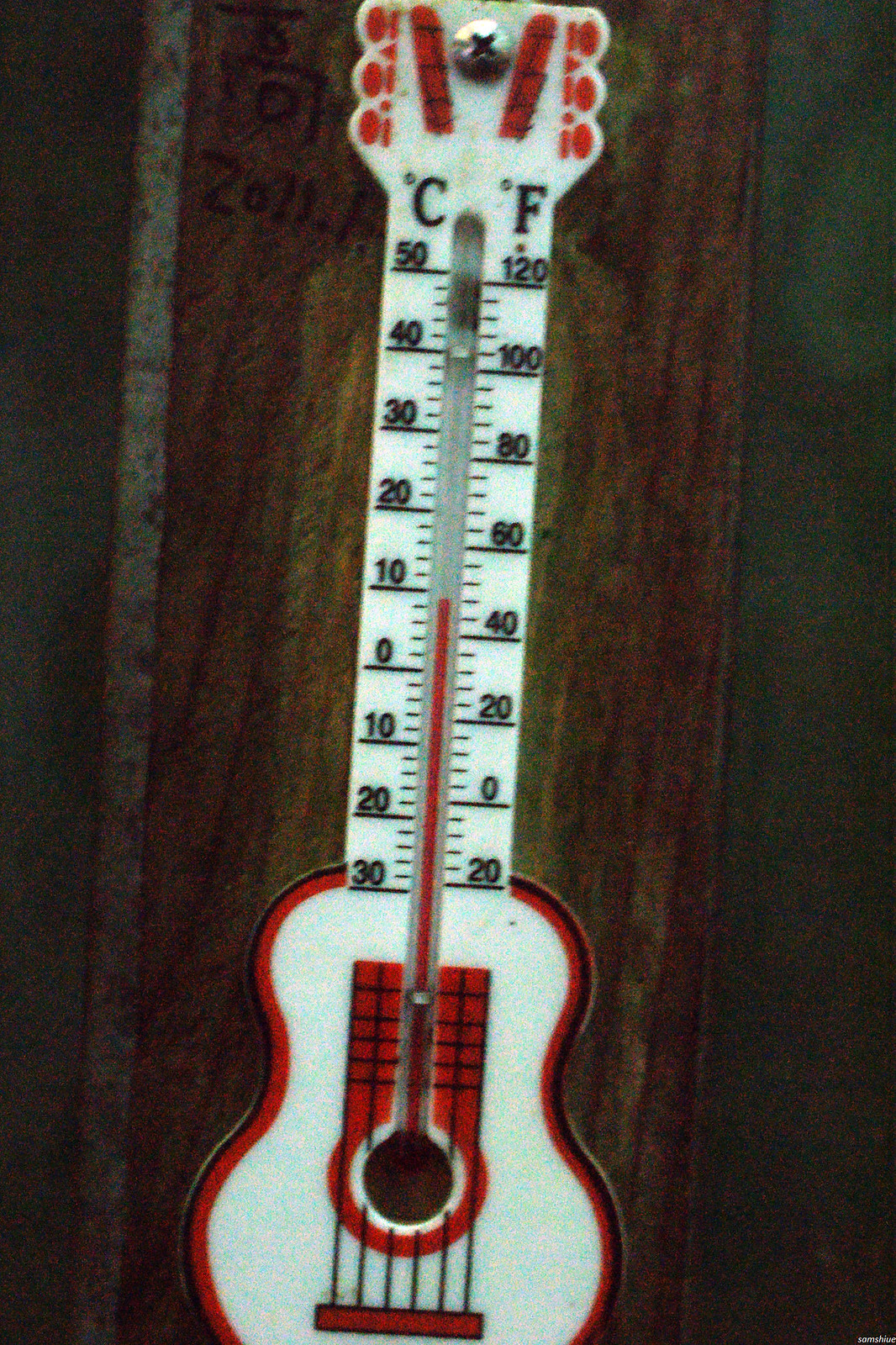The image showcases a meticulously crafted, photorealistic thermometer designed to resemble a guitar. The thermometer features a classic design, with a long, guitar-shaped body. At the base of the guitar, there's a circular, curved structure reminiscent of the guitar's body. Strings run down the center of the guitar, intersecting with a circular element that holds the base of the mercury column.

The thermometer's mercury rises straight up the middle towards the top of the guitar. The guitar's headstock, at the very top, features six tuning pegs—three on each side. Red markings in the center of this section resemble guitar studs. A silver strip at the top appears to secure the thermometer, which is mounted against a brown backboard. The backboard looks worn and may be made of cardboard, showing signs of being either nailed or stapled.

Temperature readings are displayed on both sides of the mercury column, with Fahrenheit on the right ranging from -20°F to 120°F and Celsius on the left ranging from -30°C to 50°C. The current temperature reading is about 44°F. The wooden backboard is faded, and there are some unclear marker writings in the top left-hand corner, possibly indicating a date or other inscriptions.

The entire setup is against a dark green backdrop, which adds contrast but makes certain details slightly challenging to discern.